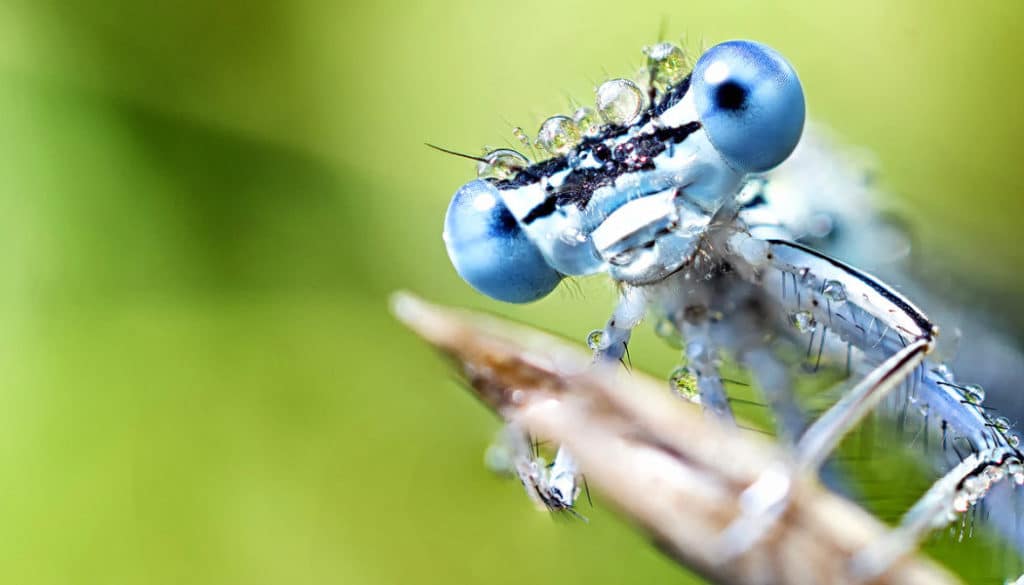Against a blurred light green background, an extreme close-up captures an intricately designed piece of jewelry mimicking an insect. The insect has an oblong head with two large, bulging blue compound eyes positioned on either side. Each compound eye features dark spots, with the left spot closer to the center and the right spot seemingly facing the viewer. Atop the insect's head, four prominent clear droplets, along with a few smaller ones, add an element of dewy realism. The face of the insect is adorned with a purple and black spot, resembling the wings of a butterfly, contributing to its ornate design.

The body of the insect, primarily blue with a black bat-like spot on the face, is complemented by its silver legs. These silver legs are delicately wrapped around an unidentifiable, light-brown object that resembles a leafy material. The legs are further detailed with black stripes and tiny hairs, adding to the intricacy of the design. The background gradations of light and dark green, with darker shades on the left, provide a contrasting yet harmonious backdrop that draws attention to the beautifully crafted insect.